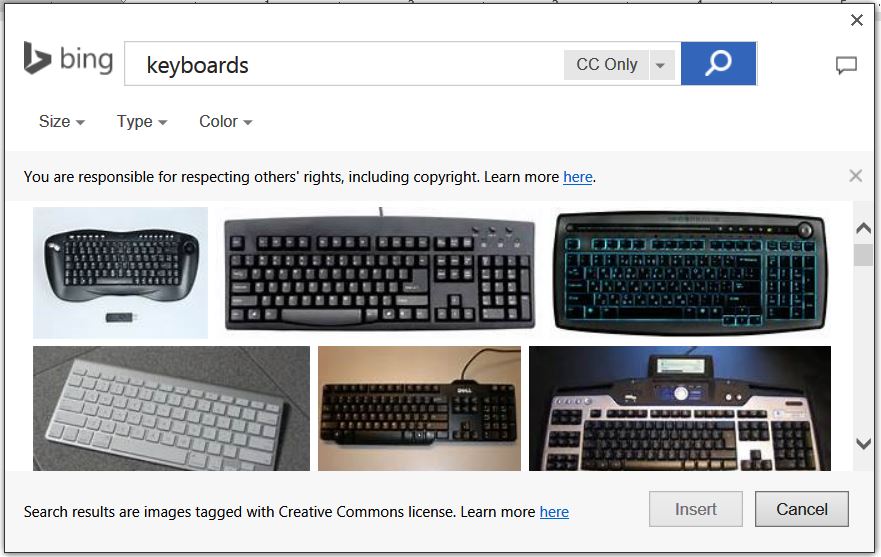**Detailed Caption of the Image:**

The image depicts a screenshot of a Bing search results page, showcasing its interface and layout in great detail. The overall page has a distinct gray border.

**Header Section:**
- At the top-left corner, there is the Bing logo and the word "Bing" displayed in gray letters, accompanied by a grey Bing emblem directly to its right.
- Next to the logo is a prominent, gray-bordered search bar containing the search term "keyboards" in black text.
- On the right end of the search bar, there are several interactive elements: a small, dark gray, gray-bordered rectangle labeled "CC ONLY," a small white line following it, a tiny gray square box with a downward pointing gray arrow, and a blue, rectangular search button with a magnifying glass icon inside.
- An 'X' icon for closing is situated at the top-right corner of this header section, with a dedicated box for entering questions or comments.

**Subcategories Section:**
- Below the Bing logo and search bar is a row comprising three dropdown subcategories:
  1. "Size" (capital S) with a downward arrow.
  2. "Type" (capital T) with a downward arrow.
  3. "Color" (capital C) with a downward arrow.

**Informational Band:**
- A light gray band is positioned below the subcategories, containing the black text: "You are responsible for respecting others' rights, including copyright." Following this sentence is a clickable text "Learn more here" (with "here" in blue, underlined text). To the right of this is a small, light gray 'X' icon.

**Image Results:**
- Below this informational band, six images of various keyboards are arranged in two rows, three per row:
  1. An ergonomically designed keyboard on a light blue background, with its USB connector visible below.
  2. A standard black keyboard with white keys and an apparent cord emanating from the top, indicating it is corded.
  3. A black keyboard without a visible cord, featuring blue-bordered keys.
  4. A tiny silver keyboard with white keys, displayed on a gray countertop.
  5. Another corded black keyboard, laying on a wooden table, with the cord visibly emerging from the right-hand side.
  6. A sophisticated-looking keyboard with silver fascia around the keys and additional controls, possibly a screen at the top, giving it an advanced appearance.

**Footer Section:**
- Below the keyboards, there is a section with the text: "Search results are images tagged with Creative Commons license." ("Creative Commons" capitalized). It is followed by the clickable and underlined text "Learn more here."
- Adjacent to this text are two rectangular, gray-bordered boxes with distinct background shades:
  1. A light gray box with the word "Insert" (capital I).
  2. A darker gray box with the word "Cancel" (capital C).